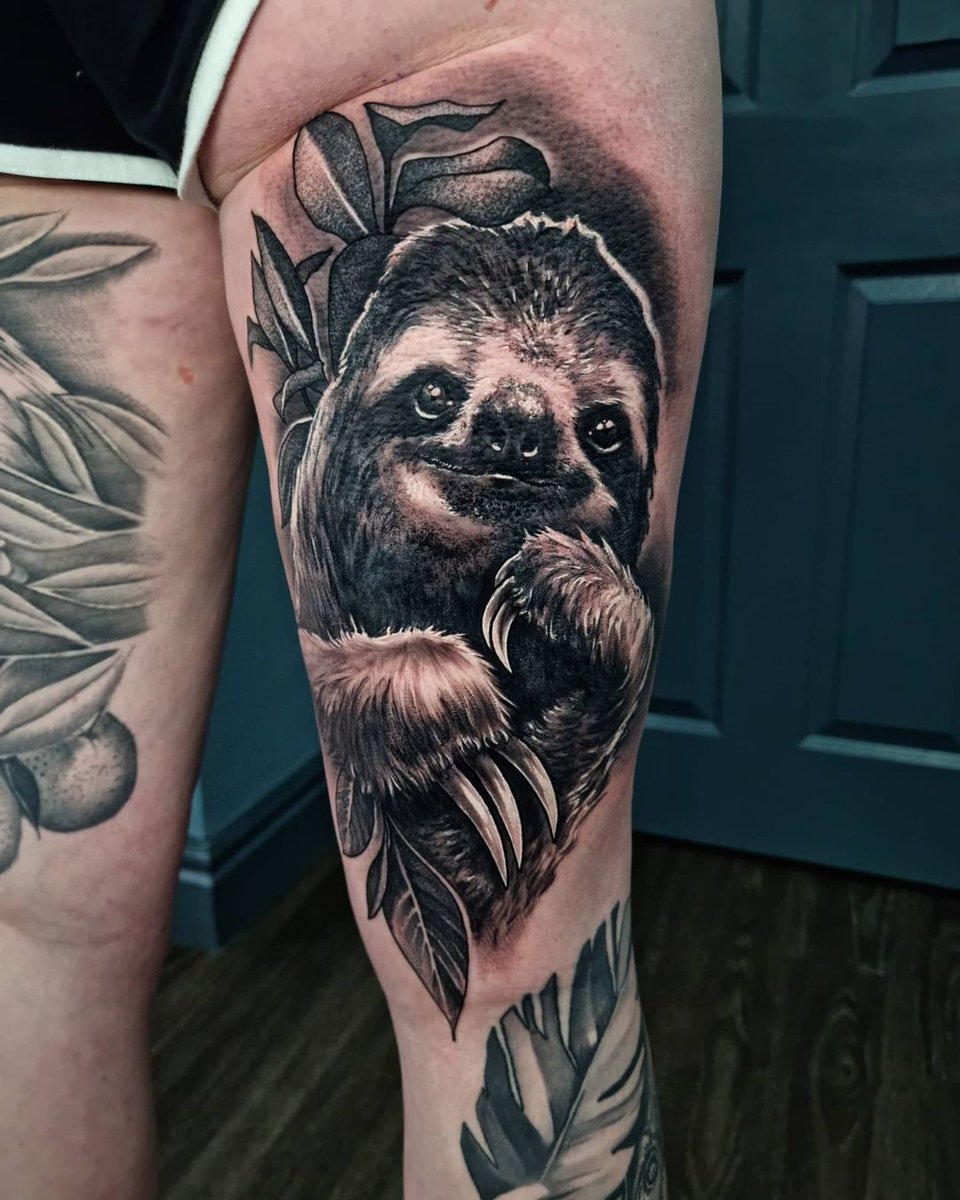This photograph captures a fresh, intricately detailed black and white tattoo of a sloth on a woman's thigh. The tattoo, located on the front upper thigh area, showcases the sloth with its paws in front of its body and a slight smile on its face. The skin around the tattoo is still slightly reddish and pink, indicating its recent completion. The artwork features impressive shading and detail, particularly in the sloth's fur, with white hair around the eyes blending seamlessly into darker regions. Above and behind the sloth, there are leaves and some dark shading that enhance the depth of the design. Below this new tattoo, there's an older black and white leaf tattoo, further adding to the intricate tattoo work on her leg. In the background, a partial view of another tattoo on the back of her other leg is visible, as well as her black shorts with white trim.